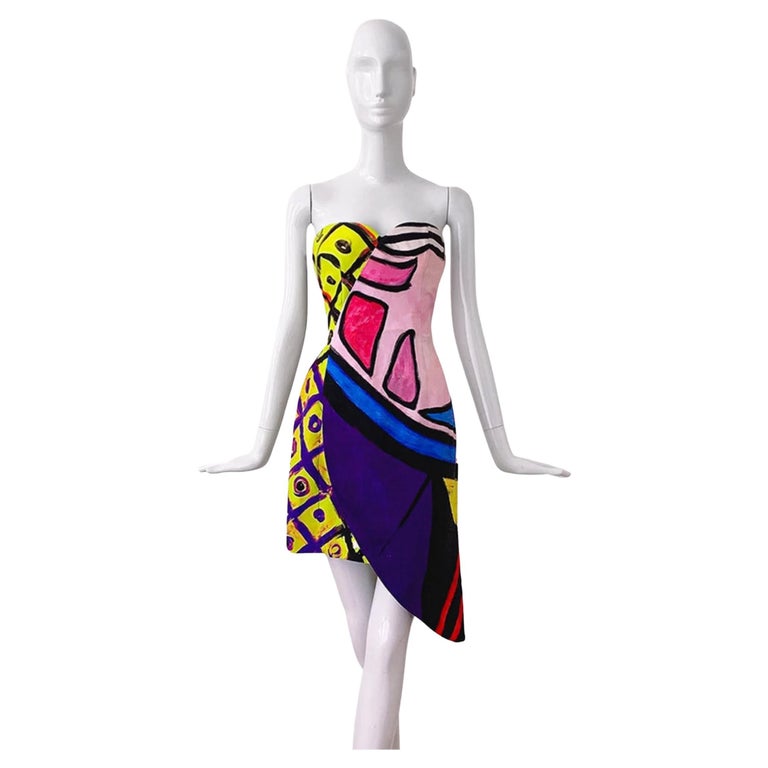In the image, a tall, slender, white mannequin stands with its legs crossed, even though it is upright. The mannequin is bald and has its arms positioned at its sides with hands flared outward. The vibrant, eye-catching dress it is wearing has a strapless sweetheart neckline and falls to about knee length. The dress features an eclectic mix of patterns and colors: the left side is adorned with yellow and purple diamond border, while the right side has a pink top with darker pink geometric shapes. Below, a strip of dark blue transitions into a predominantly dark purple lower section. Additional color accents include black and white stripes, along with red elements, creating a fashion-forward, striking visual. The dress showcases a blend of solid shapes, lines, and checkered patterns, making it a central, attention-grabbing piece in the image.